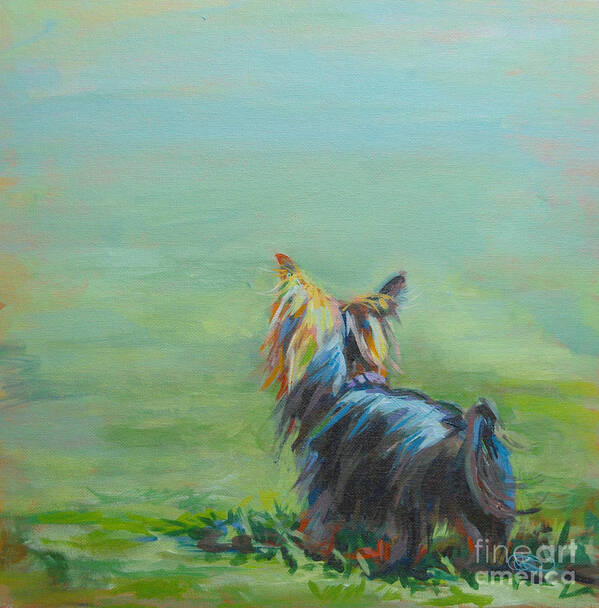This image is a vibrant and detailed painting of a small Yorkie dog, prominently featuring a Fine Art America watermark in the bottom right corner. The Yorkie, painted in an array of colors, stands in a grassy field that blurs into a mix of green, teal, and blue hues, giving an impressionistic feel to the scene. The dog, facing away from the viewer, sports a tuft of yellow fur on top of its head, which gradually darkens along its back, with blue and red streaks accentuating its shaggy coat. Pointed ears and a black tail are visible, adding to the charming depiction. The grass around the Yorkie varies slightly in height, emphasizing the dog's small stature and creating an intimate, whimsical atmosphere.